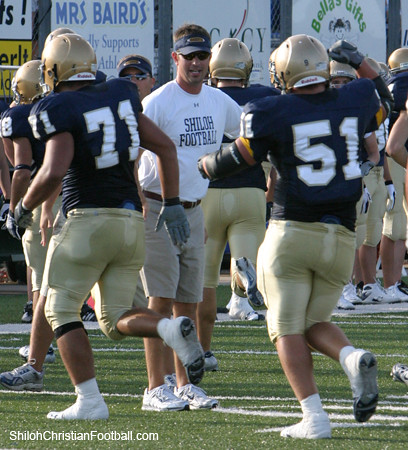The image captures an emotional moment at a football event, showcasing players as they leave the field. The photo is zoomed in and prominently features two football players wearing uniforms similar to Notre Dame's, with gold helmets, navy blue jerseys, and gold pants. The player on the left has the number 71, while the one on the right has the number 51. They are running off the field, with several more players visible in the background. A man, presumably part of the coaching staff, stands by in white sneakers, shorts, a white t-shirt that says "Shiloh Football," and black sunglasses. He is greeting the players with his hands out, appearing to give them high-fives. In the lower part of the image, a credit reads "ShilohChristianFootball.com," and sponsors' banners are visible in the stadium backdrop.